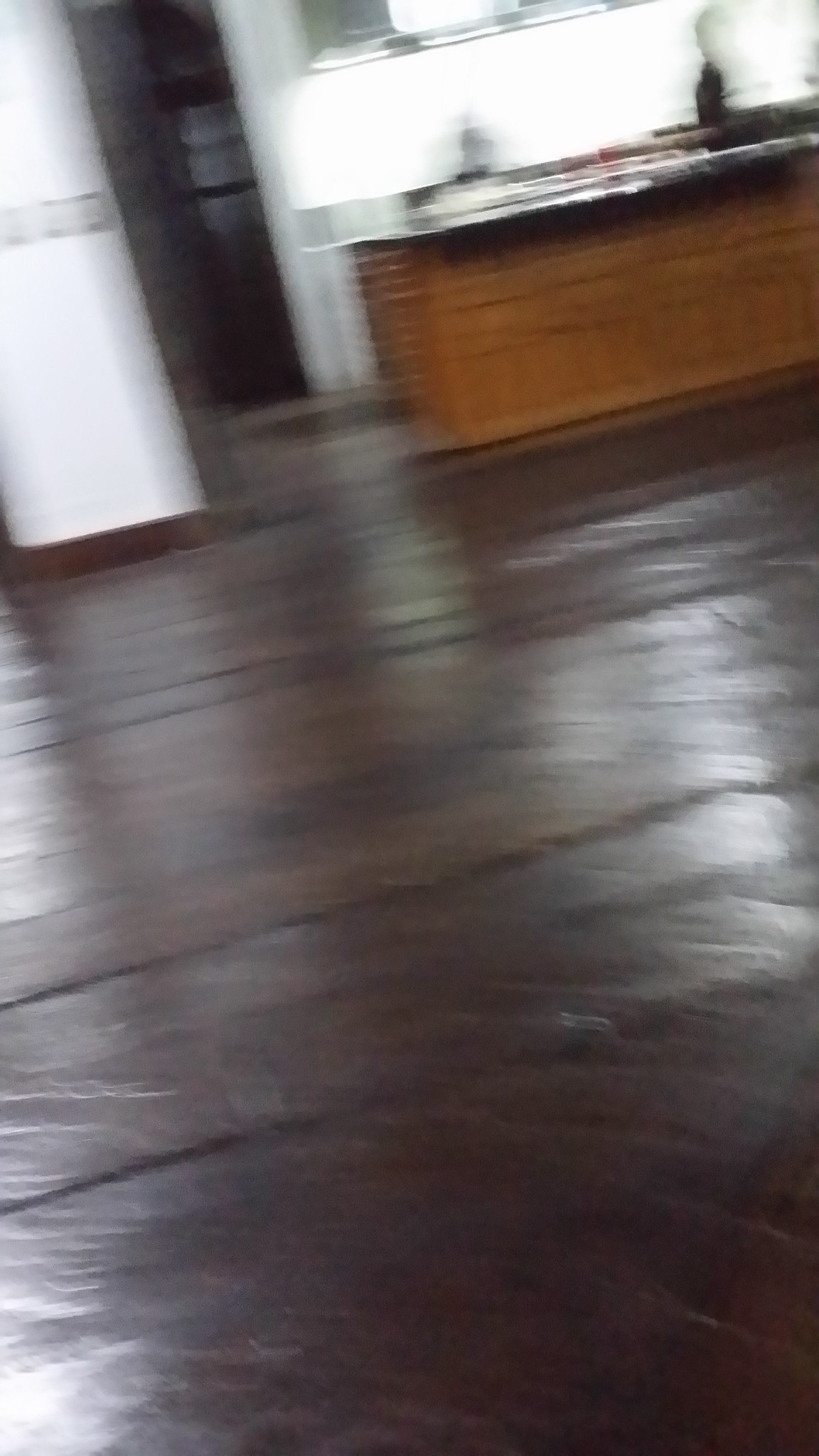The image depicts an extremely blurry photo of what appears to be an empty kitchen. The scene is angled, likely due to the camera being tilted while in motion, suggesting the photo was taken hurriedly or accidentally. The dominant feature is a dark brown hardwood floor with a subtle sheen from reflected light. On the far left, there's a partially visible stained-glass door with a white interior and brown edges, hinting at an exterior exit. Adjacent to this door is an open, dark area, possibly another door receding into the background.

On the right side of the image, the white wall stretches upwards, reflecting considerable light. The wall is capped by a sliver of a window with a silver frame, only just visible at the top of the picture. Below this is a light brown desk or countertop with a dark brown surface that also catches some light. This area likely forms part of the kitchen, given the countertop's positioning and the scattered objects upon it, though their details are obscured by the blurriness.

Together, the elements — the wooden trim around the doors, brown cabinetry visible on the right, and empty floor space — compose a snapshot of an unfurnished, modestly lit kitchen, distinguished primarily by its muted color palette and the tilt of the incomplete frame.